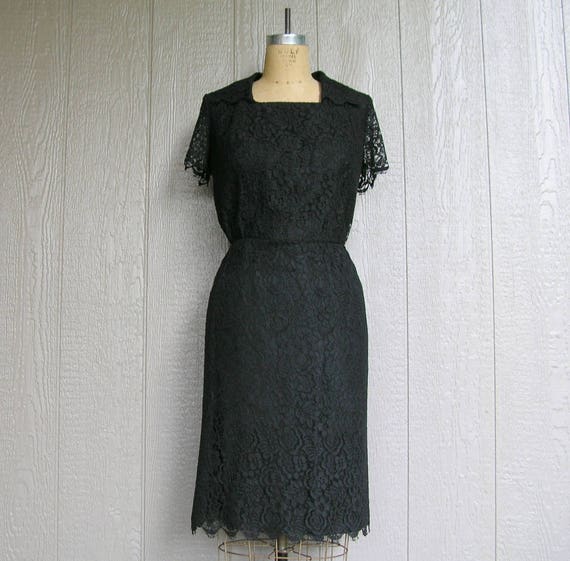The image features a sleek and elegant black dress displayed on a headless and armless mannequin form with a yellow, skin-toned torso. The dress, which falls just below the knees, has a sophisticated design marked by a square neckline and short sleeves made of delicate black lace. The main body of the dress is plain, possibly with a satin base under a lace overlay, and is slightly gathered at the waist to enhance its fit. The hemline is subtly adorned with a zigzag pattern, adding a touch of unique flair. This ensemble stands against a background that combines different elements—predominantly a paneled wall that looks grayish with vertical wooden lines, giving it a well-maintained appearance with light reflecting off parts of the surface. The overall setting suggests a formal presentation, likely within a boutique or display shop.